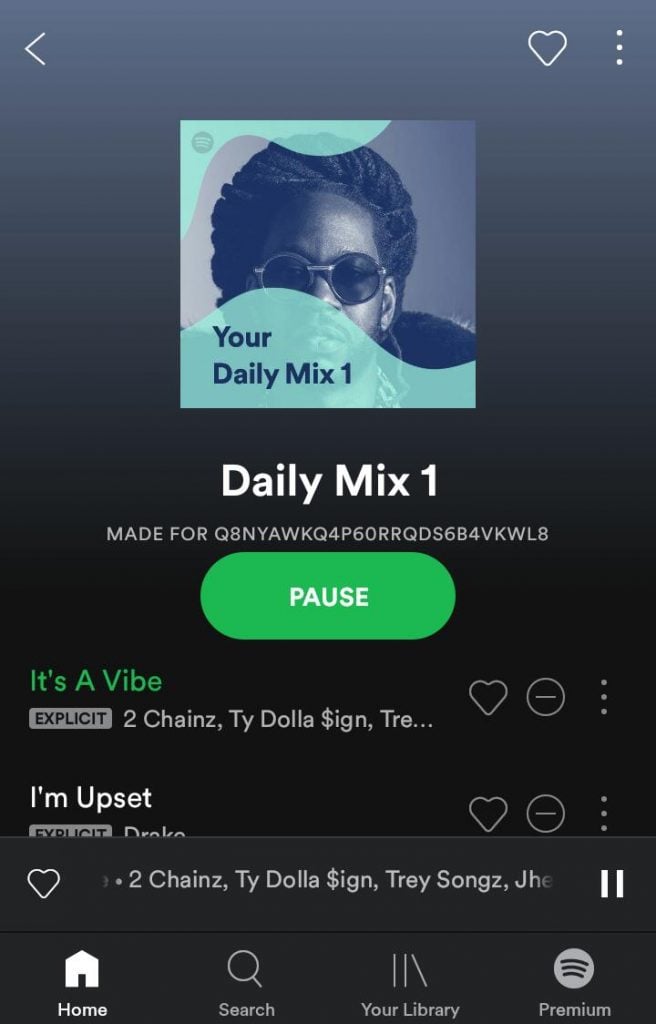This is a detailed descriptive caption for the given image:

---

The image is a cropped screenshot from a mobile device, showcasing only an application window. The top part of the screen features a square image of a black male wearing brown sunglasses, overlaid with the text "Your Daily Mix," suggesting a personalized musical playlist. The playlist is titled "Daily Mix 1," with the title prominently displayed. Below the title, a large green pause button indicates that music is currently playing. Specifically, the song "It's a Vibe," marked as explicit, is the top song listed and is actively playing. At the bottom of the screen, there are four navigation icons: a home icon depicted as a house, a search icon illustrated with a magnifying glass, a library icon represented by three lines resembling a stack of books on a shelf, and a premium icon portrayed as a white circle with three curved lines inside it. The overall image focuses solely on the application interface without displaying any physical phone details or the top edge iconography typically seen on the device screen.

---